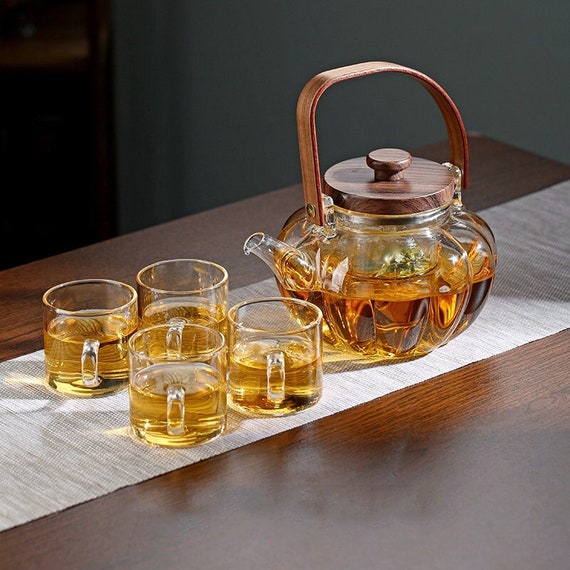This color photograph captures a serene tea set arrangement on a dark wooden table. At the center of the table lies a white fabric table runner. To the left, four clear glass teacups, each with handles pointing towards the viewer, are halfway filled with an amber liquid, presumably tea. The transparent cups, showcasing the light brown substance, are neatly organized. On the right, a clear glass teapot, half-filled with the same amber tea, features a distinctive wooden lid and a brown leather handle. Centered within the teapot is a clear basket containing tea leaves. The background reveals a plain white wall and a door, enhancing the simple elegance of the setting.